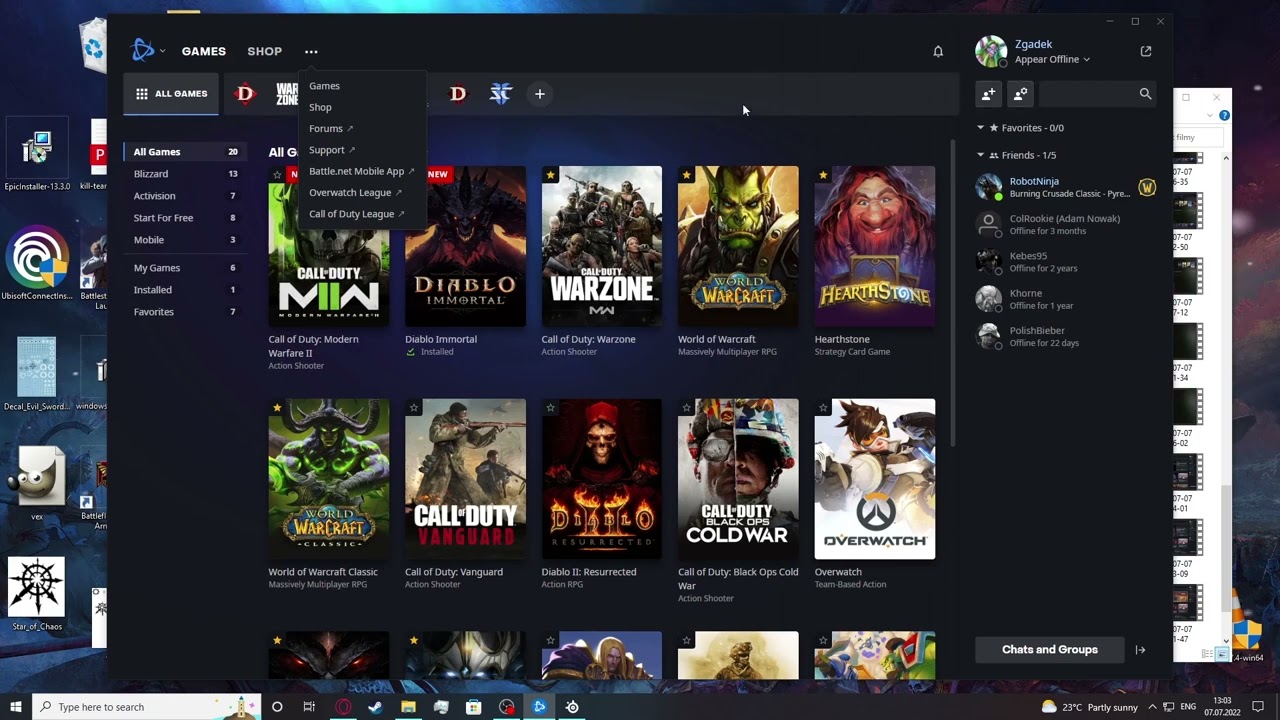A detailed caption for the image:

The image displays a computer home screen, showcasing a vibrant desktop background adorned with an array of application shortcuts. Among the visible icons, there is a trash can, a PDF viewer, Ubisoft Connect, and several other shortcuts, indicating a preference for gaming-related applications. Ubisoft Connect, in particular, is a notable feature as Ubisoft is renowned for its video games.

Central to the image is an open application, presumably a game management or launcher program, displaying a library of games. One of the highlighted games, "Devil Mortal," is already installed, as indicated by the installation status beneath its icon. The interface of the application shows a selection of games available for downloading or purchasing. On the left side of the application, there are various menu options, and on the right side, there is a friends list detailing online status and durations of inactivity.

In the background, another window appears to be open, likely containing videos, suggesting that the user might be a streamer or content creator. The overall setup, with multiple gaming and media-related applications, strengthens the notion that the user is deeply engaged in gaming and possibly streaming activities.